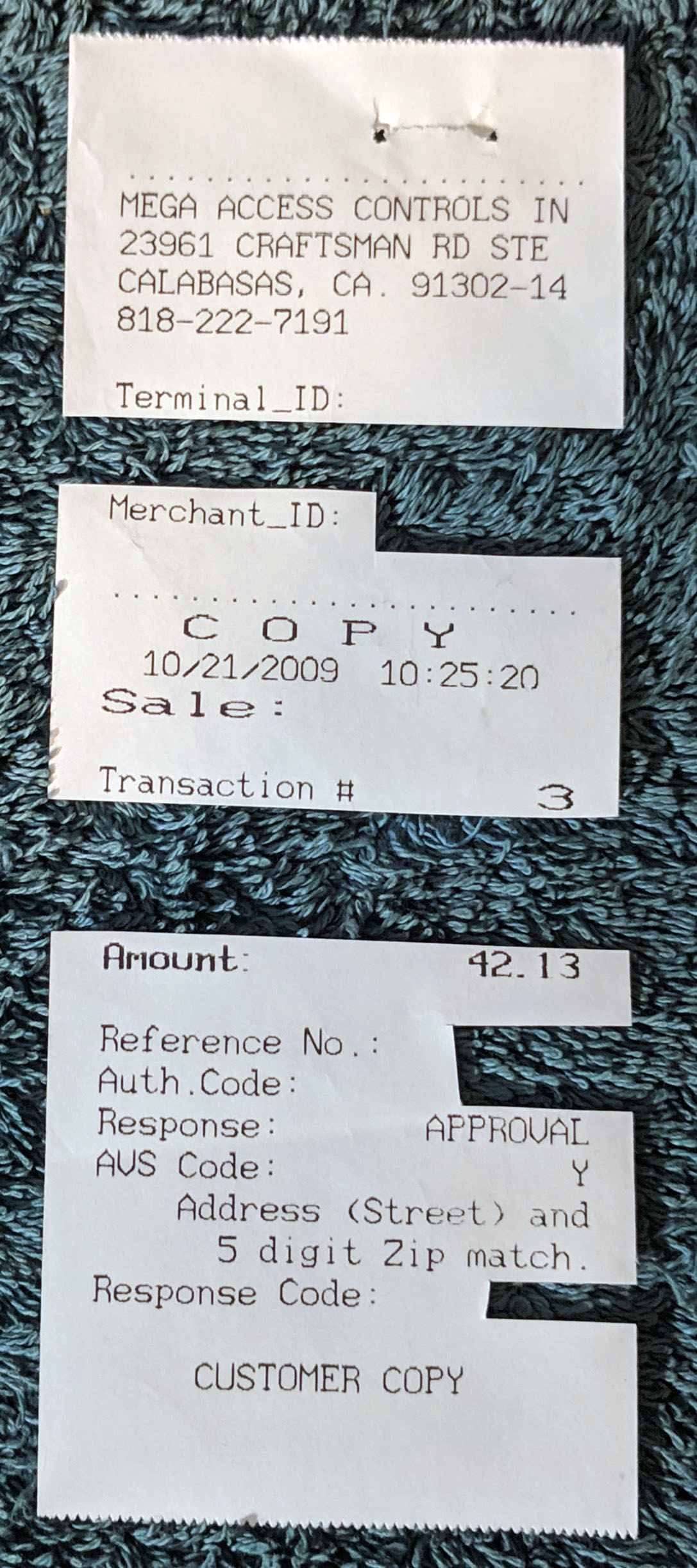This is a close-up photograph of a receipt that has been cut into three distinct sections, all lying vertically on a blue shaggy carpet. The top section of the receipt, which features a perforated edge and staple marks, reads "Mega Access Controls, 23961 Craftsman Road, Ste, Calabasas, California, 91302-14" along with the phone number "818-222-7191." It also includes the Terminal ID. 

The middle section of the receipt displays "Merchant ID," followed by "Copy," the date "10-21-2009," the time "10:25:20," "Sale," and "Transaction Number 3," along with a small segment cut off from the top right corner. 

The bottom section outlines the amount "$42.13," with other fields such as the reference number, authorization code, and response code being cut out. This part of the receipt is also marked as the "Customer Copy." The three sections are visibly laying on a blue-gray carpet with a long nap, providing a clear view of the details and cuts made to the receipt.